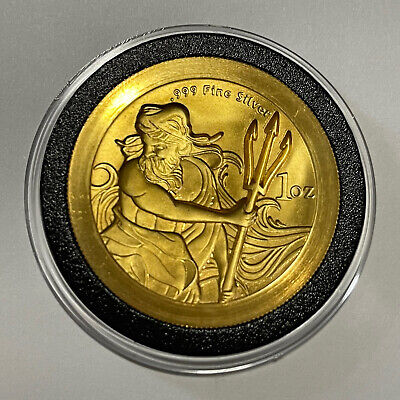The image features a photograph of a gold coin enclosed within a clear plastic case, which appears to be set on a gradient grey background. The coin has a detailed design with multiple elements: the outer edge is silver with a black speckled ring inside. At the very center, there's a prominent gold section featuring a muscular, bearded Viking-like figure holding a pitchfork or a serpent-like staff, reminiscent of mythological deities such as Zeus. The Viking is surrounded by waves in the background. The coin has raised lettering noting its specifications, including ".999 Fine Silver" at the top and "One Ounce" inscribed on the gold section. The coin is cushioned by a foam edge within the plastic casing, ensuring its protection and display.